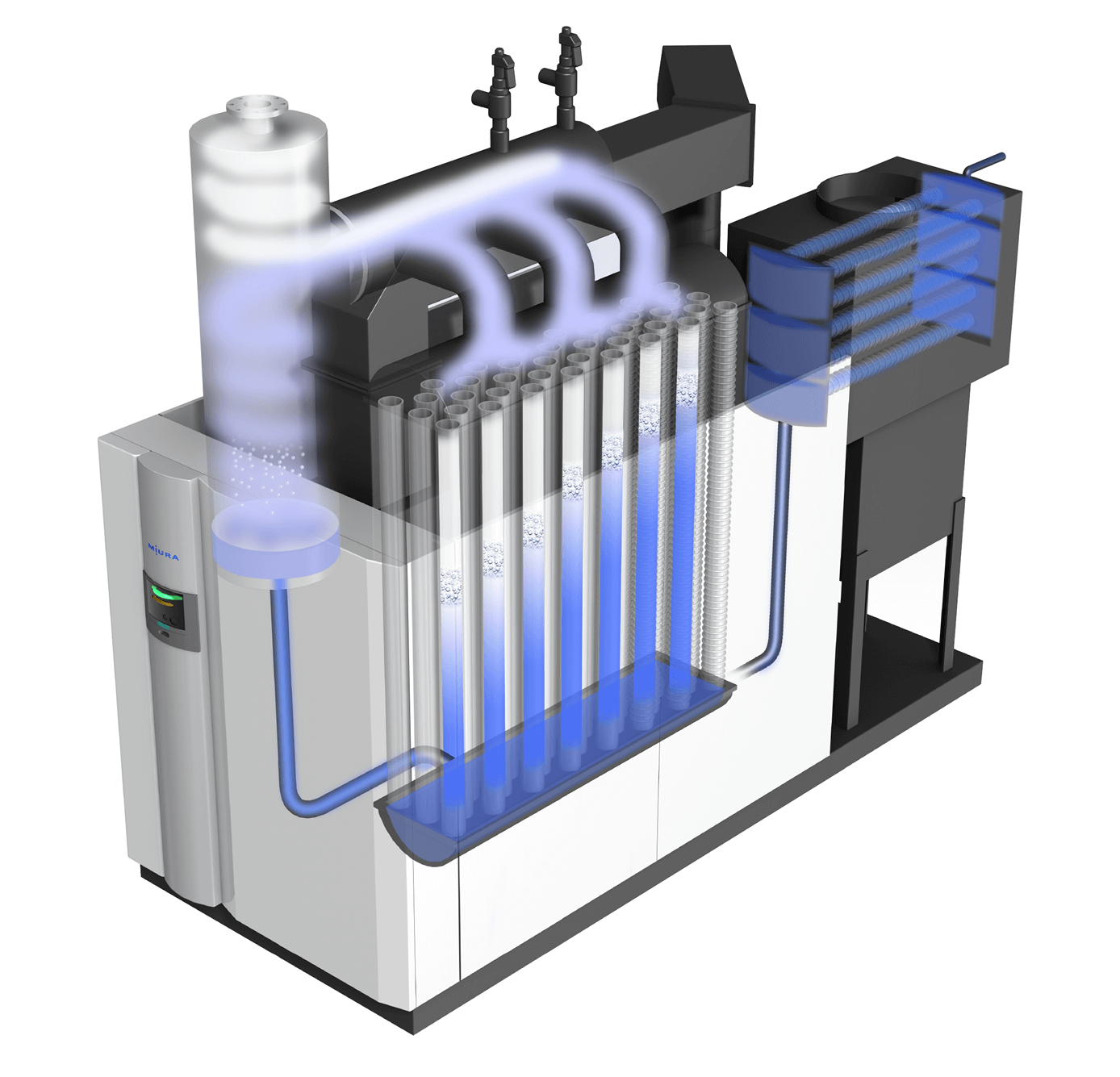The image showcases a detailed and intricately designed machine, depicted as a digital line drawing or 3D model set against a plain white background. The machine, primarily white and square-shaped, features a front panel with an unreadable text display, a green indicator light, and a small opening, likely intended for a cup to collect filtered water or chemicals. The central body of the machine houses a tall cylinder and an array of interconnected tubes, through which a blue liquid or chemical appears to circulate. These tubes, some visible through an opaque section of the machine, are filled with the blue substance, illustrating the filtration or pumping process. At the top of the machine, there are two handles possibly used for operating the machine, and on the far right, a black box with a rotatable handle or pulley system, suggesting further control mechanisms. Overall, the image likely represents a scientific contraption or filtration system with visible chemical flow, although its exact purpose remains unspecified.